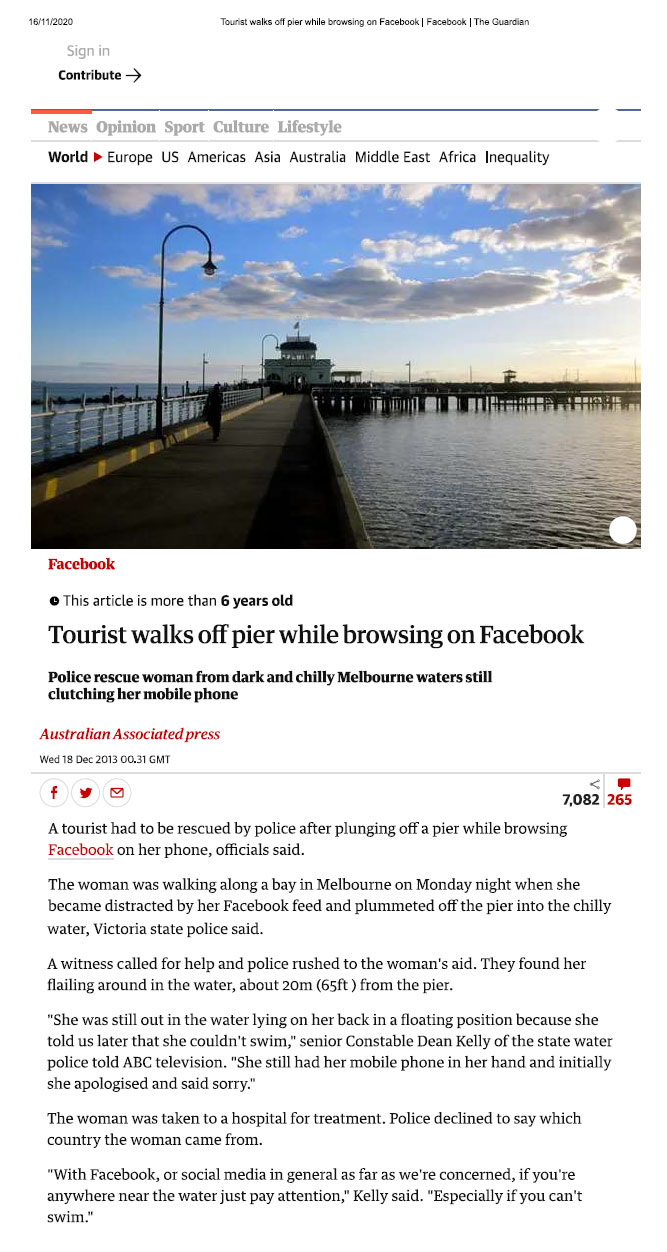This image captures a detailed view of a news article on a website. The webpage features a white background in the top left corner with the date "16/11/2020" displayed in black text. Central to the top of the page is a headline reading, "Tourist Walks Off Pier While Browsing on Facebook," written in black font, followed by vertical lines partitioning sections. The title is flanked by "Facebook" and "The Guardian," also in black text.

Below the date, near the top right, there is a gray "Sign in" link. Directly underneath this, a bolded black text reads "Contribute" with an arrow pointing to the right. A black horizontal line extends across the width of the page with a small open space about an inch from the right edge. Just below this line on the left side is a short red line about two inches long.

Further down, the navigation menu appears in gray text, listing "News," "Opinion," "Sport," "Culture," and "Lifestyle" from left to right. This is followed by another gray horizontal line. Beneath this line, in bolded black text, it says "World," next to a sideways red triangle with its tip pointing to the right. Adjacent to this, the categories "Europe," "US," "Americas," "Asia," "Australia," "Middle East," "Africa," and "Inequality" are listed out.

The central image of the article shows an outdoor scene of a person walking down a pier. The background includes a small white boat dock floating on water that varies in shades of light and dark blue, and the sky is dotted with clouds.

Below this photograph is the main story's title in bold red text, "Facebook." Directly underneath, the text indicates that "This article is more than six years old," and the main headline is restated: "Tourist Walks Off Pier While Browsing on Facebook." The article body consists of about three or four paragraphs elaborating on the incident.